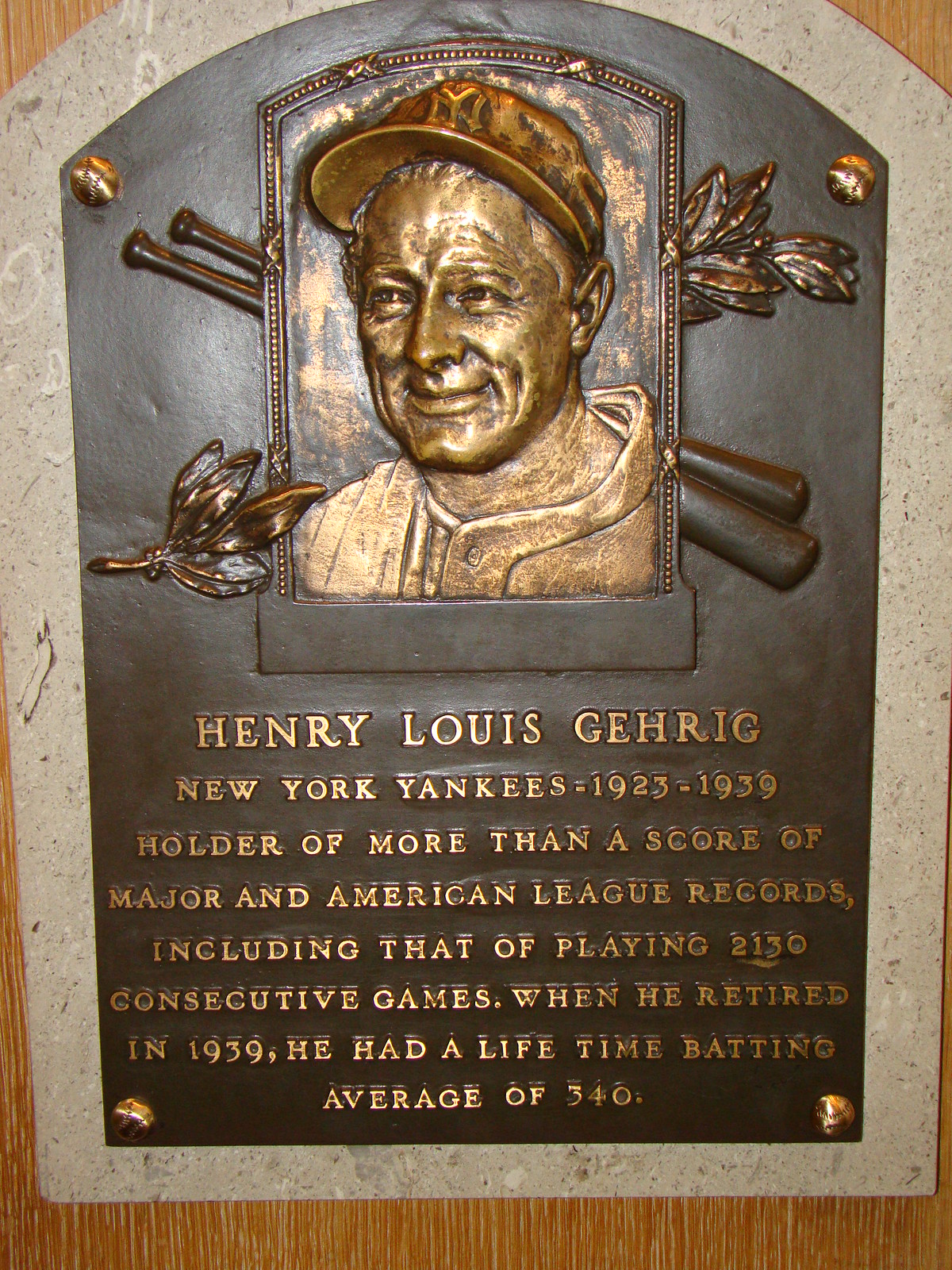The image features a detailed bronze plaque dedicated to the legendary baseball player Henry Louis Gehrig of the New York Yankees, who played from 1923 to 1939. Central to the plaque is a bronzed, textured portrait of Gehrig, depicted smiling and looking to the left while wearing a New York Yankees cap. Positioned diagonally behind the portrait are two crossed baseball bats, their ends visible at the top left and bottom right of the plaque. Decorative leaves extend diagonally from the top right and bottom left corners. Surrounding the portrait are four small bronze baseballs, one in each corner of the plaque.

The inscription on the plaque highlights Gehrig’s historic achievements: "Henry Louis Gehrig, New York Yankees, 1923-1939. Holder of more than a score of Major and American League records, including that of playing 2,130 consecutive games. When he retired in 1939, he had a lifetime batting average of .340." 

The plaque itself is mounted on a light marble base, which in turn is set against a dark wooden surface, creating a striking contrast that accentuates the bronze and gold details.